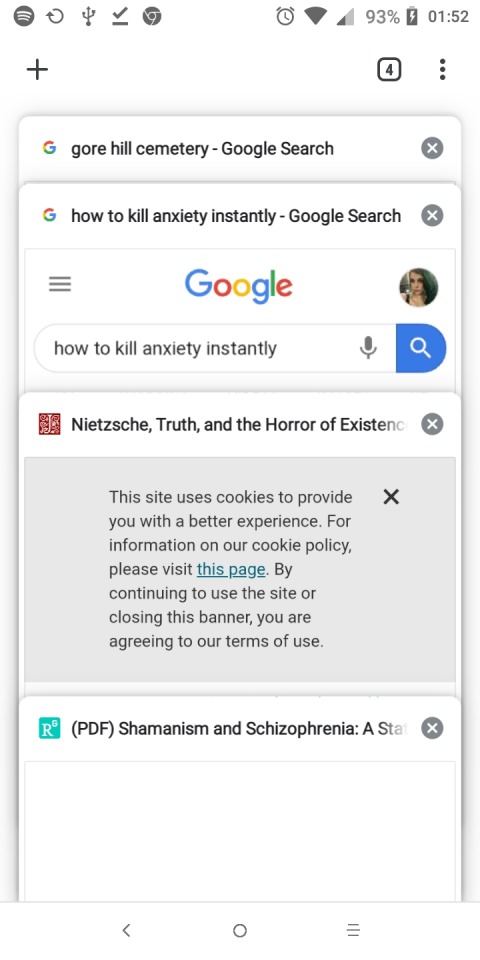The image depicts a cell phone screen with a white background. In the top left corner, we see standard cell phone icons, similarly mirrored on the top right. These include the clock showing 01:52, a full Wi-Fi signal, a cellular signal with two out of five bars, and a battery icon at 93% with a lightning bolt indicating charging. 

Beneath this status bar, on the top left, a plus icon is displayed. On the top right, there's a unique icon: a black outlined square containing the number four, indicating multiple open tabs, next to three vertical dots suggesting more options.

The screen reveals several stacked search pages, with each page partially visible. The top visible page shows a Google search for "Gore Hill Cemetery." This page features the multicolored Google "G" logo on the left side and an "X" button on the far right to close the tab.

Further down, the next search page shows a query for "how to kill anxiety instantly." In the middle of this page, the word "Google" is prominently displayed in the brand’s signature colors. To the right is a small circular profile picture. The search field containing the query is accompanied by a microphone icon and a blue search button with a magnifying glass icon in white.

The following page features an article titled "Nietzsche, Truth, and the Horror of Existence," with a red square and white detailing on the right. Below the article title, there's a gray notification bar indicating that the site uses cookies. It includes a teal, underlined link to the site's cookie policy and text explaining that continued use or closing the banner implies agreement with the terms of service.

The final visible tab shows a search for a PDF titled "shamanism and schizophrenia." 

This detailed view of the cell phone screen captures various ongoing searches and essential status indicators, reflecting both the user's concerns and their browsing patterns.